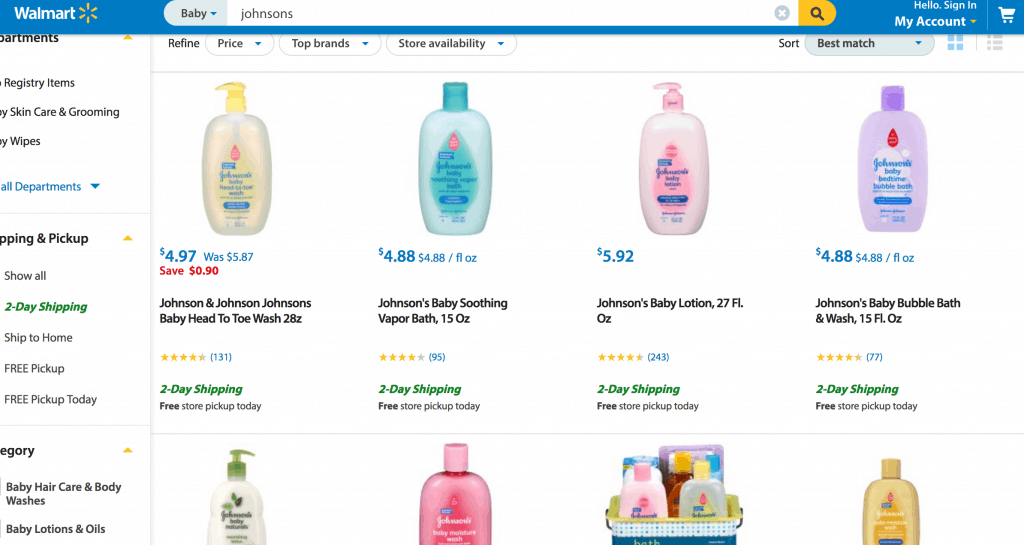The image displays a webpage for shopping baby products on Walmart's website. The Walmart logo, identifiable by a small snowflake icon, is located in the top left corner. The search bar has the query "baby Johnson's." On the top right, options to "hello, sign in to my account" and access to the shopping cart are visible.

On the left side, there's a menu with categories such as departments and shipping. The main content area focuses specifically on baby products, more precisely Johnson's brand items. Displayed across the webpage are eight products, but only the first four are fully visible due to the image cutoff.

The listed baby products include:
1. Johnson's Baby Head to Toe Wash priced at $4.97.
2. Johnson's Baby Soothing Vapor Bath priced at $4.88.
3. Johnson's Baby Lotion priced at $5.92.
4. Johnson's Baby Bubble Bath and Wash, available in a 15 fluid ounce bottle.

The webpage reflects the common sentiment that parents often purchase baby products based on perceived cuteness or quality.